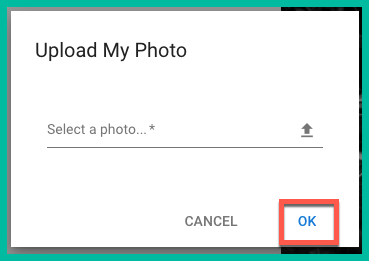A detailed view of a screen capture taken from a website, showcasing a user interface designed for photo upload. The background of the image is predominantly white, enhancing the clarity of the interface elements. The screenshot itself is vertically oriented, and is framed by a thin to moderately sized green border. Nested within this green border is another border, predominantly gray, that surrounds most of the internal interface, except for a black section that outlines the right, top, and bottom edges, creating a U-shaped pattern of black.

Inside this bordered area, on the left-hand side, there is a prompt that reads "Upload my photo". Beneath this prompt, a search box is positioned, displaying the text "Select a photo" and accompanied by an arrow, suggesting that the user can scroll through options. Two buttons are also visible at the bottom of this interface: a "Cancel" button, and an "OK" button. The "OK" button is blue and distinctly marked with a red rectangle around it, emphasizing its importance for finalizing the selection.